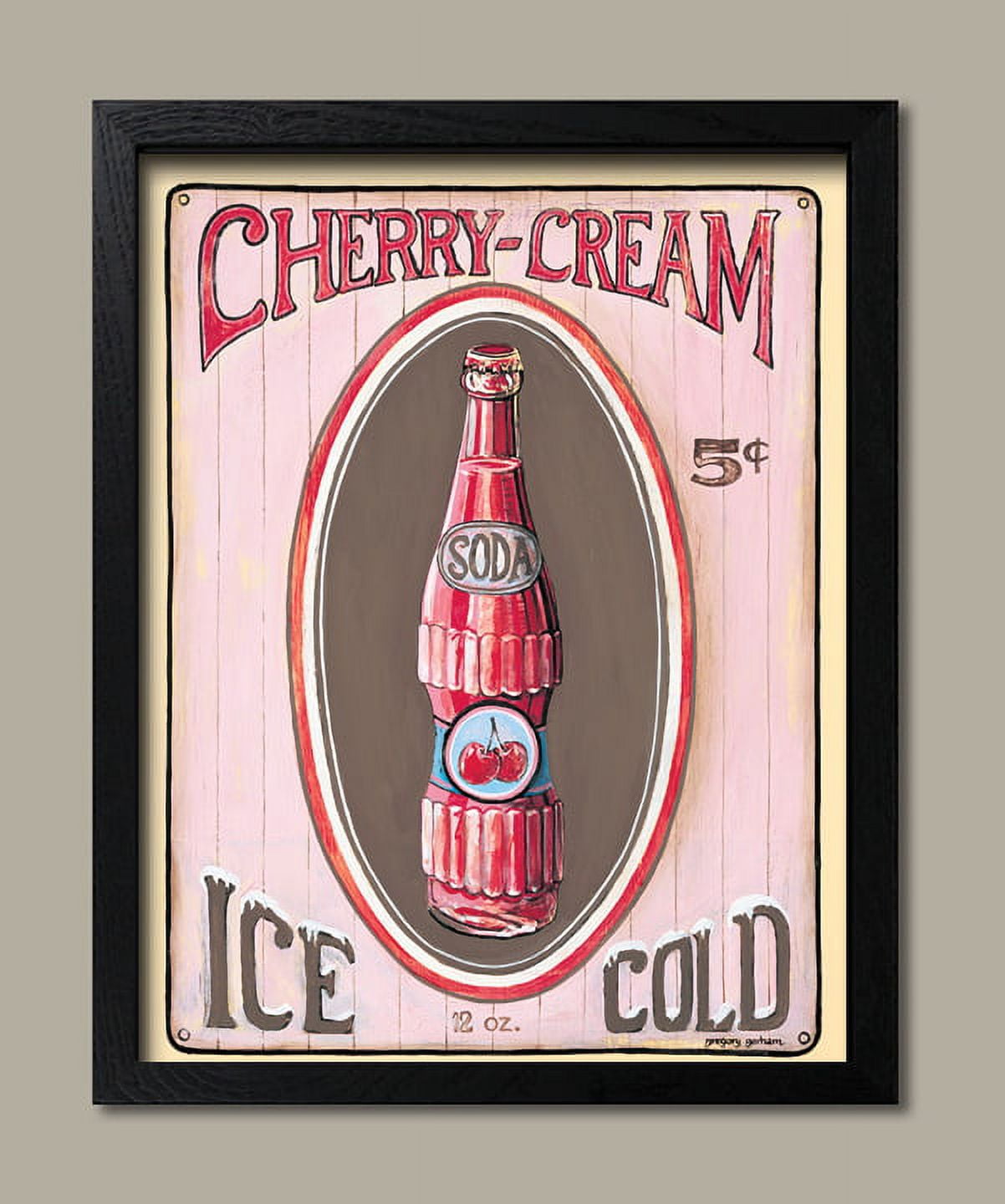The image features a painting of a vintage soda advertisement framed within a black wooden frame, mounted on a beige wall. The painting has a soft yellow border and depicts an old metal sign with circular mounting holes in each corner. Across the top of the sign is an arched red text that reads "Cherry-Cream." Below the text, in the center, is a tall oval containing a detailed painting of a vintage glass soda bottle. This bottle, with a red label and a depiction of cherries in the middle, has the word "Soda" on its neck. Surrounding the bottle is a series of nested ovals: the inner one is brown, the middle one is white, and the outer one is red. To the right of the ovals is the price, marked as "5¢". Below the ovals, the words "Ice Cold" are split with "Ice" on the bottom left and "Cold" on the bottom right, appearing to be topped with ice or snow. Additionally, the sign indicates that the bottle contains 12 ounces of soda.